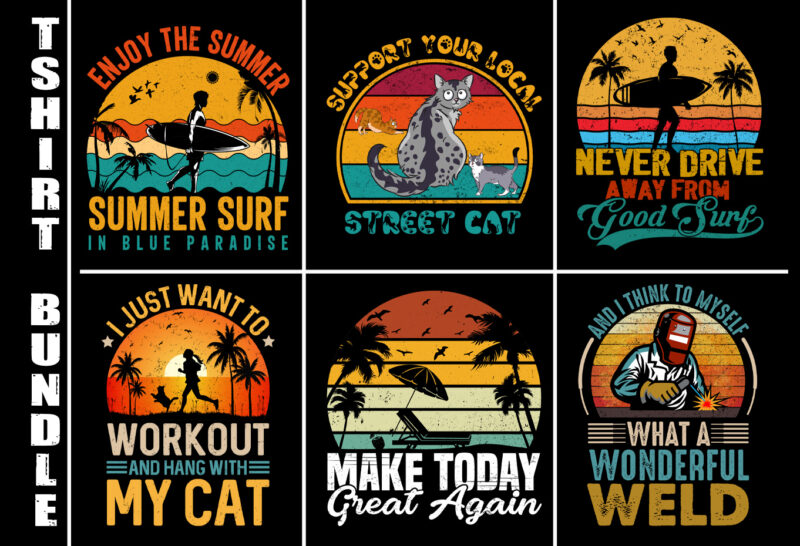This image is an advertisement for a t-shirt bundle consisting of six colorful and vibrant t-shirt motif designs, all set against a black background. On the left side, vertically aligned text reads "T-SHIRT BUNDLE." The six designs share a summer and surfing theme, with a playful twist on outdoor and pet-related activities.

1. **Top Left**: "Enjoy the Summer, Summer Surfing, Blue Paradise" — This graphic shows a surfer holding a surfboard, walking by the waves with a backdrop of palm trees in vibrant sunset hues.
   
2. **Top Middle**: "Support Your Local Street Cat" — This design features multiple cats, centered around the text, spotlighting a community-focused cat theme.
   
3. **Top Right**: "Never Drive Away from Good Surf" — Another surfing-themed image with a surfer holding a surfboard, flanked by palm trees and seagulls, capturing the essence of beach life.
   
4. **Bottom Left**: "I Just Want to Work Out and Hang with My Cat" — This motif depicts a person running with their cat amid a picturesque sunset, blending fitness and pet companionship.
   
5. **Bottom Middle**: "Make Today Great Again" — Accompanied by images of a lounge chair, beach umbrella, palm trees, and birds in the sky, this image encourages relaxation and seizing the day.
   
6. **Bottom Right**: "And I Think to Myself What a Wonderful Weld" — Featuring a welder with a welding hat and gloves, actively welding metal, this design uniquely celebrates the art of welding.

Each t-shirt design offers a distinct yet cohesive representation of summer life, from surfing adventures and beach relaxation to feline love and welding craftsmanship.